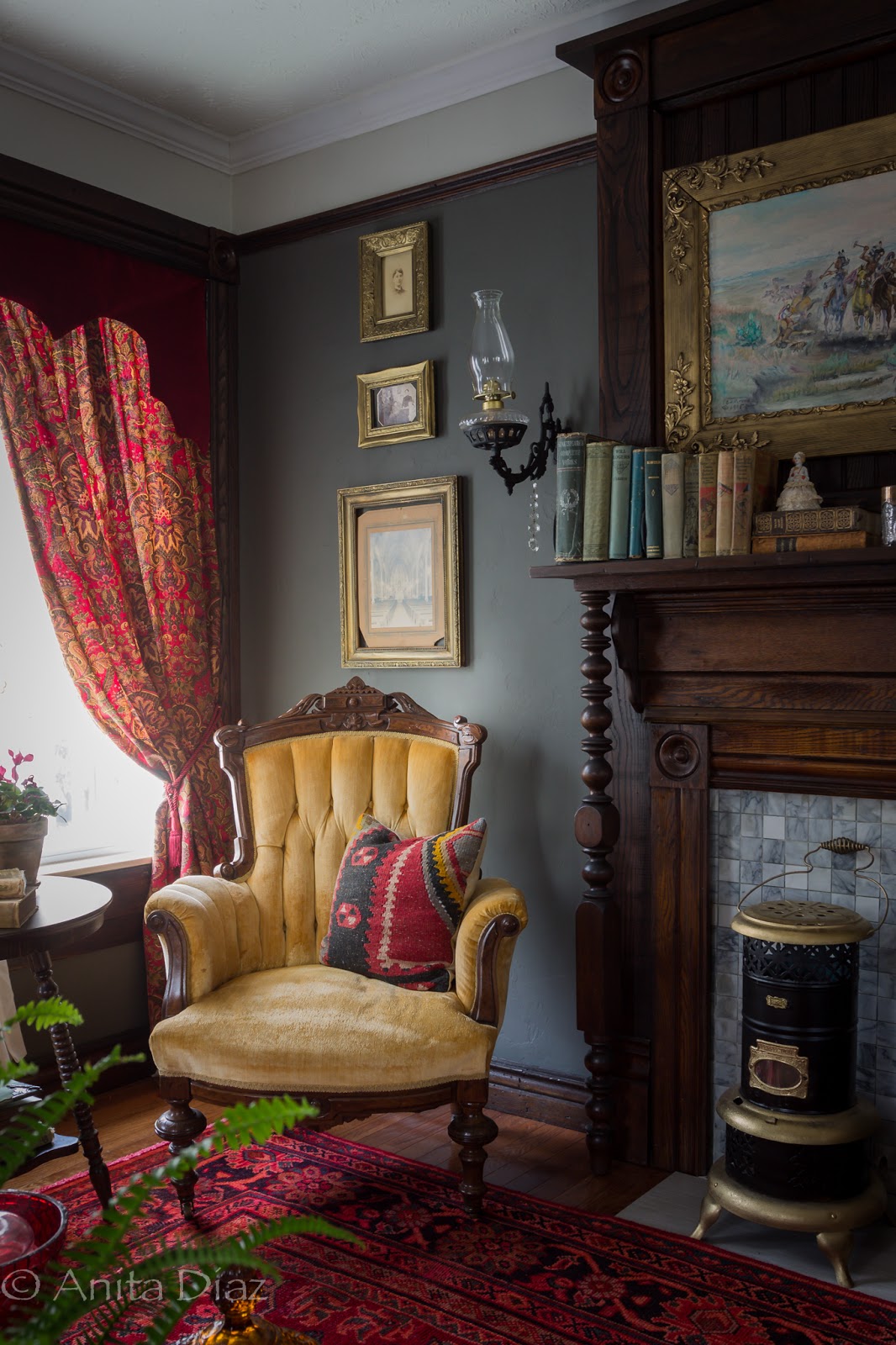This real-life photograph, copyrighted by Anita Diaz, captures an elegantly decorated sitting room corner, evoking an Art Deco charm. Central to the space is a fireplace adorned with an antique wood heater, framed by numerous books—about 12 to 13—meticulously arranged on the mantel. Above the mantel hangs a framed piece of fine art, likely a scene inspired by the colonial period. To the left, the wall features a glass light fixture and several picture frames, possibly three, though their details are indistinct. The walls are painted a dark sage green, contrasting beautifully with the white ceiling.

A standout piece in the room is a plush, vintage gold chair with a woven fabric, accompanied by a throw pillow. Enhancing the seating area is a small side table topped with a potted plant, complemented by a fern that adds greenery to the space. The flooring is polished hardwood, partially covered by a red and black paisley area rug. The room is bathed in daylight, streaming through custom red and gold paisley curtains pulled aside, revealing a window. This thoughtfully curated room, with its blend of vintage elements and rich, warm tones, offers a cozy reading nook that feels both quaint and refined.